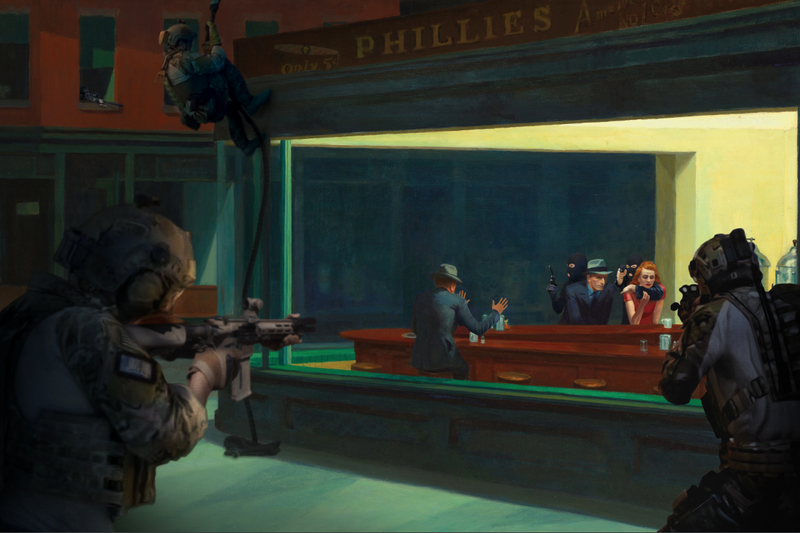The painting vividly captures a tension-filled scene inside a bar, prominently marked with the name "Fillies" in yellow letters. The composition offers a glimpse both inside and outside the establishment through large windows, where two men in army fatigues are positioned with rifles aimed into the bar. Outside, another officer is seen descending a rope. 

Inside the bar, which is brightly lit by natural light, the central focus is on captives and their captors. A man in a suit and hat, with his back against the wall and hands raised, is seated on a barstool, clearly terrified. Opposite the bar, a dramatic confrontation unfolds: a woman with red hair and a matching red dress is held hostage by a masked man, his arm menacingly around her neck. Nearby, another suited man, also wearing a hat, is under the threat of a second armed and masked assailant.

The detailed painting features a vivid color palette ranging from greens and reds to yellows and blacks, enhancing the clarity and intensity of the scene, as the hostages fear for their lives.